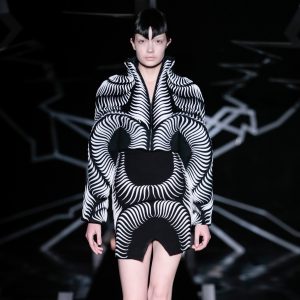The photograph depicts a light-skinned woman standing against a dark black background, centrally aligned in the square frame. She has strikingly short, black hair, parted in the center and styled to point towards the bridge of her nose, bearing a resemblance to Spock from Star Trek. Her face is bare of makeup, with shaved eyebrows that have been meticulously drawn in with pencil, and she stares forward with a blank, emotionless expression.

Her outfit is a unique and abstract design featuring black and white stripes reminiscent of zebra patterns. It is a long-sleeved garment with a short skirt that ends high above the knees, leaving her legs bare. The garment includes an enormous white circle at the waist, resembling arches, complemented by a black pouch-like feature, and finishes with additional white and black arches at the skirt's hem.

The background is adorned with silver and white lightning bolt-like streaks, resembling spider legs or webs radiating out from behind her, enhancing the surreal and abstract nature of the scene. The woman's outfit, combined with her stark expression and bold hairstyle, creates a visually striking and avant-garde composition.